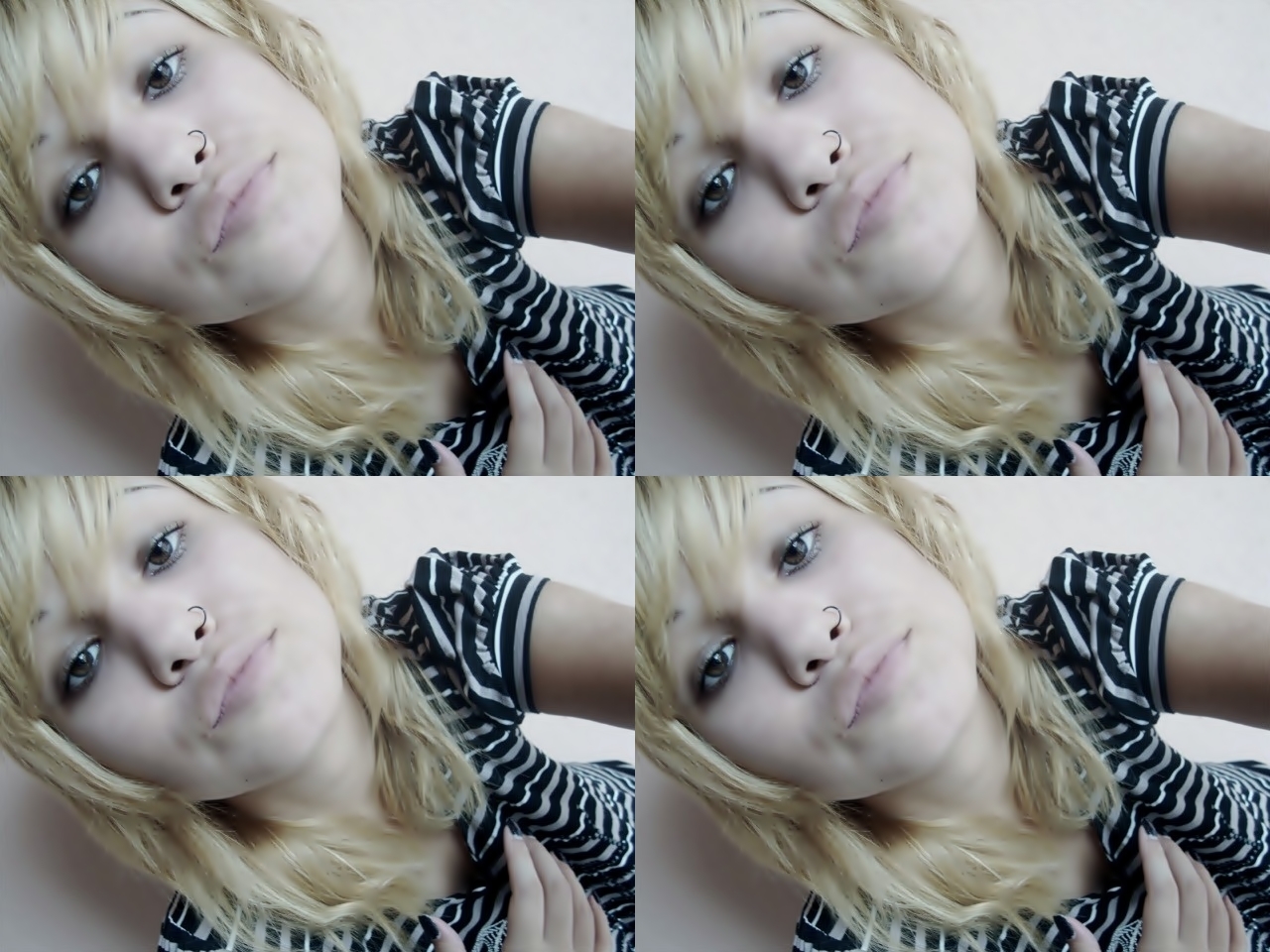The image is a collage of four identical slightly off-center selfies of a young, Caucasian girl with light brown eyes and blonde hair. Each photo, tilted approximately 40 degrees to the right, shows her with her head in the upper left and her mid-stomach in the lower right. She has thin eyebrows, partially covered by bangs, and wears black and white horizontal striped short-sleeved shirt. The girl, looking directly into the camera with a subtle, half-pursed smile, sports a nose ring on her left nostril. She is wearing makeup, including eyeliner that accentuates the sparkle in her eyes. Her right hand, with nails painted black, rests casually on her middle, and she is positioned against a wall.